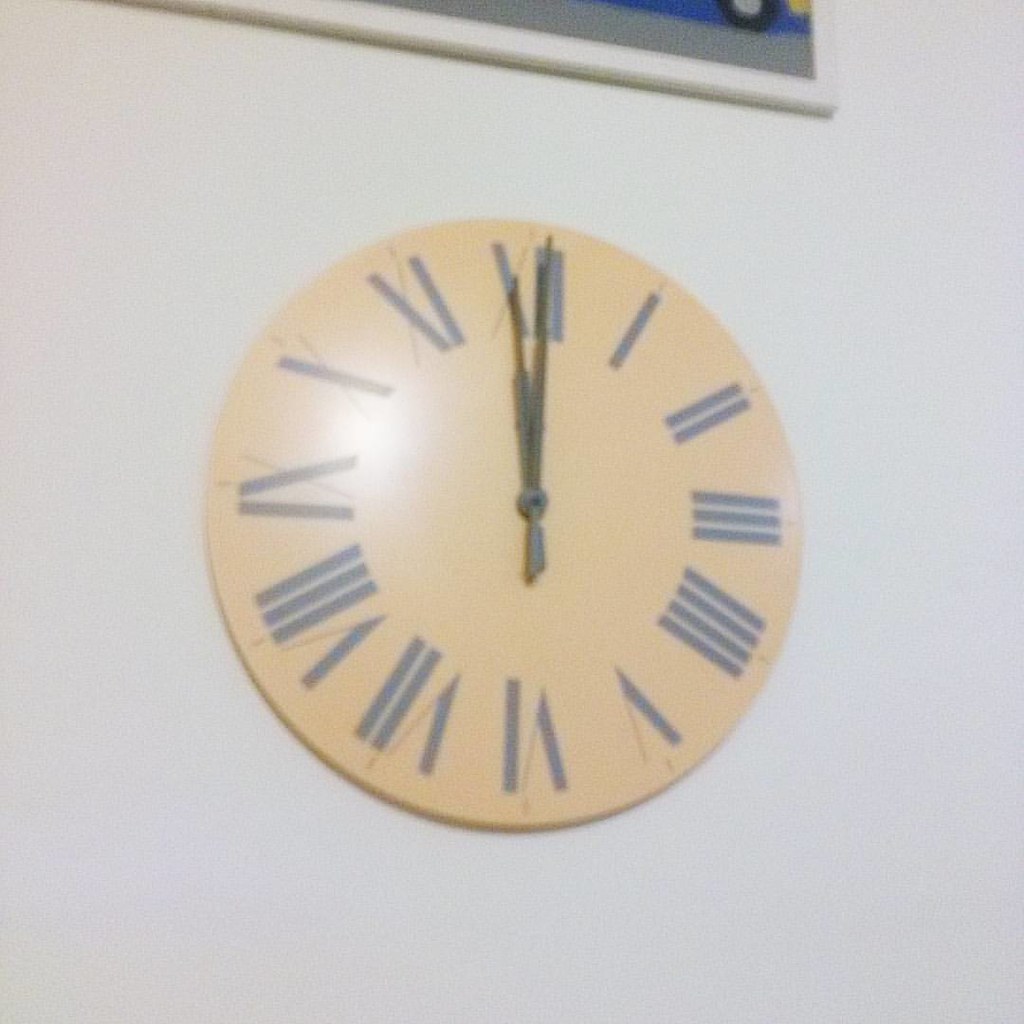This indoor photograph, slightly angled, captures a simple, round clock mounted on a white wall. The clock, with a light peach or butter yellow background, prominently features Roman numerals for its numbers. The time displayed is approximately 12:01, with both the hour and minute hands just off vertical alignment. The clock is unframed, with no glass covering the hands, which appear to be dark-colored, possibly plastic or metal. A bright light from the upper right casts a shadow and some glare on the left side of the clock face, particularly around the nine o'clock position. In the upper portion of the image, part of a thin white frame of another artwork is visible, hinting at a larger picture just out of sight. The overall photograph is very light, slightly grainy, and somewhat out of focus.